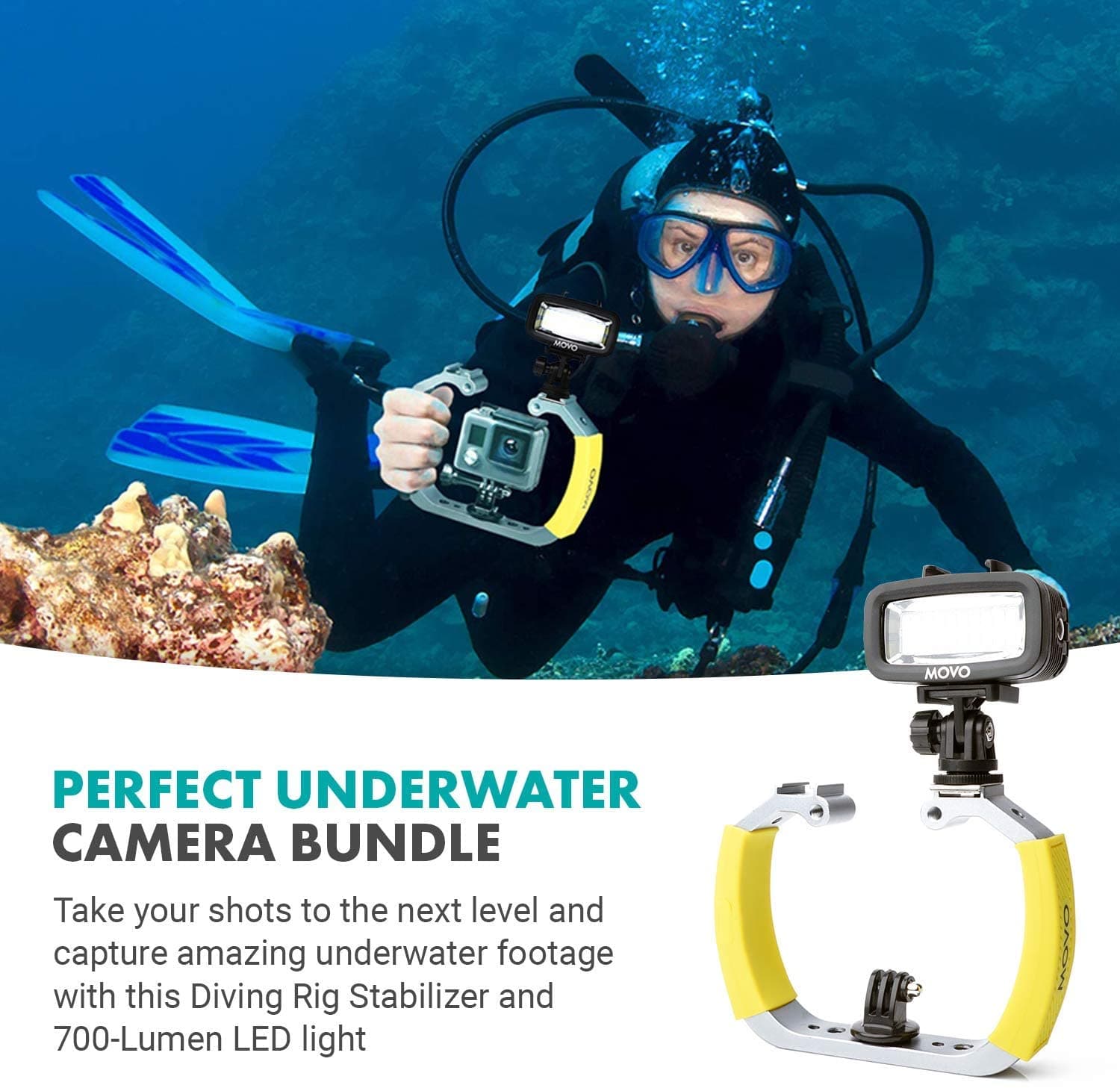The image showcases an underwater advertising photograph, possibly taken from a magazine or online. It features a female scuba diver in a black wetsuit with blue-rimmed goggles, bubbles escaping from her scuba apparatus. She is equipped with a scuba tank on her back, with tubes extending to her mouthpiece. In her right hand, she holds a sophisticated underwater camera rig, which includes a stabilizer and a 700-lumen LED light. This rig features a U-shaped yellow foam handle apparatus designed for stabilizing a GoPro camera. The diver’s turquoise flippers, which are dark blue on the inside, add a splash of color to the deep blue underwater scene. On the coral-strewn bottom left of the image, text in turquoise letters reads "Perfect Underwater," followed by "Camera Bundle" in black letters. Below that, an advertising copy states, "Take your shots to the next level and capture amazing underwater footage with this diving rig stabilizer and 700 lumen LED light." To the right of the text is a detailed product image of the yellow-handled camera stabilizer and LED light setup, designed for capturing perfect underwater shots.